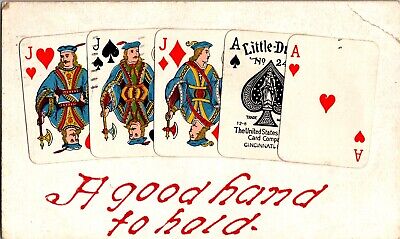This image depicts an antique deck of playing cards arranged in a fanned-out, full house formation on a cream-colored, distressed background. The cards, showing signs of age and wear, include the Jack of Hearts, Jack of Spades, Jack of Diamonds, Ace of Spades, and Ace of Hearts, aligned from left to right. The designs on the cards evoke a classic 19th-century aesthetic, enhancing their vintage charm. Beneath the cards, in elegant red handwriting, the phrase "a good hand to hold" is inscribed, adding a nostalgic touch to the scene. The background itself features subtle creasing and distress marks, contributing to the overall antique feel of the tableau.